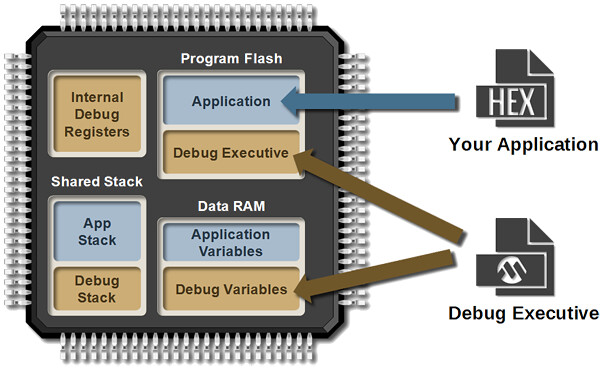This detailed, computer-generated illustration depicts a microchip-like structure. The central figure is a dark black box with rounded silver spirals resembling the bindings of a spiral notebook on all four sides, indicative of a computer chip's design. Within this structure, there are seven distinct squares and rectangles, each filled with text and varying in color, primarily blue and brown.

In the central areas, the labeled components include "Internal Debug Register," "Application," "Debug Executive," and "Debug Stack." Notably, the "Application" and "Debug Executive" are interconnected and segmented within a section labeled "Program Flash." To the far right, there's an icon of a black piece of paper with the word "HEX" on it, accompanied by a blue arrow pointing towards the "Application" square. Below this, another blue arrow points from the "HEX" icon to the two "Debug Executive" sections, indicating a flow or relationship among these components. The image succinctly represents various elements related to software debugging within the confines of a microchip layout, highlighting key areas and their interconnected functions.